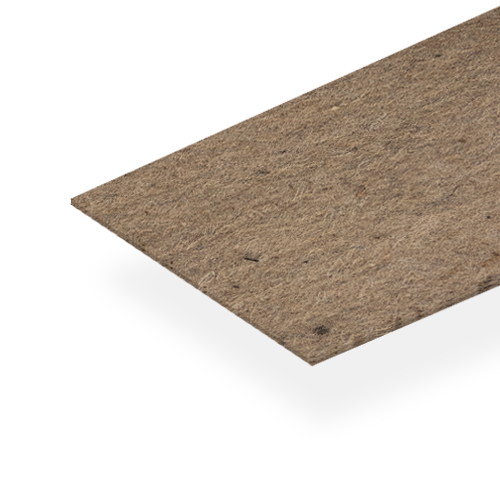This image depicts a long, rectangular mat made of thick fabric, placed on a bright white surface. The mat boasts a primary brown color punctuated by small patches of darker brown and lighter, yellowish-brown spots in various shapes, including circular patterns and tiny lines. The fabric displays a textured appearance with some fibers protruding from it, contributing to its rugged look. The mat has well-defined edges and casts shadowing underneath, although whether this shadowing is real or digitally edited is unclear. The mat, about 1 cm thick, extends from the right side of the image to the middle, with the rest of its length cut off from view.